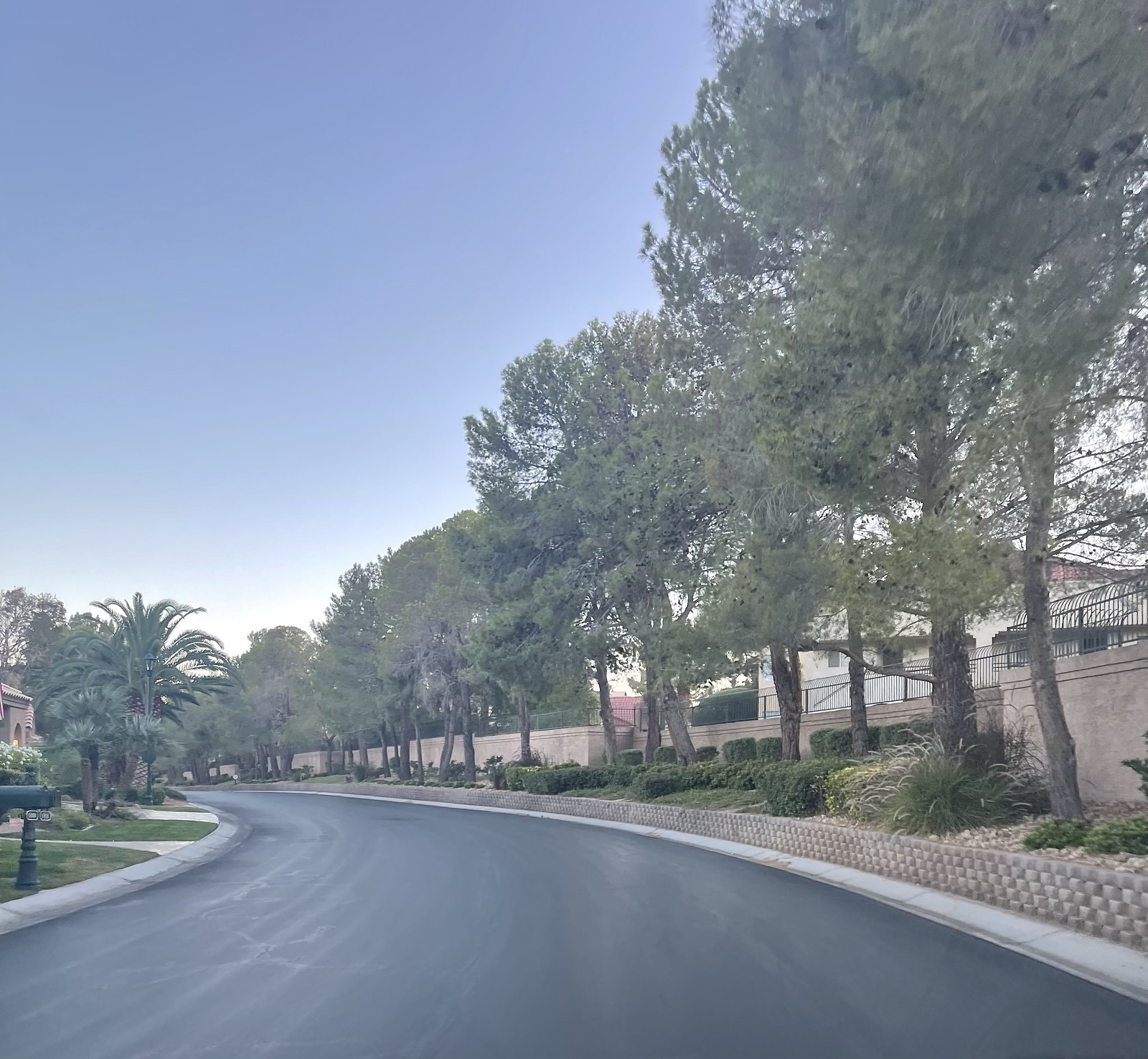This photograph captures a wide, dark paved road devoid of traffic lane markings, suggesting it winds through a housing development. Flanked by trees on both sides, the scene exudes an air of suburban tranquility. On the right side, a meticulously crafted stone border, approximately one to two feet high, delineates the road from the landscaped area behind it, which features gravel, grass, and manicured shrubs. Just beyond the trees, houses are partially visible, secured by iron or metal fencing. To the left, the road is accompanied by multiple driveways, a black mailbox, and several palm trees that partially obscure another house. The line of trees on the right side follows the curvature of the road, leading the eye deeper into the scene. The sky overhead is a pristine blue, adding to the serene ambiance. In the distance, a house with a distinct pinkish-colored roof punctuates the background.